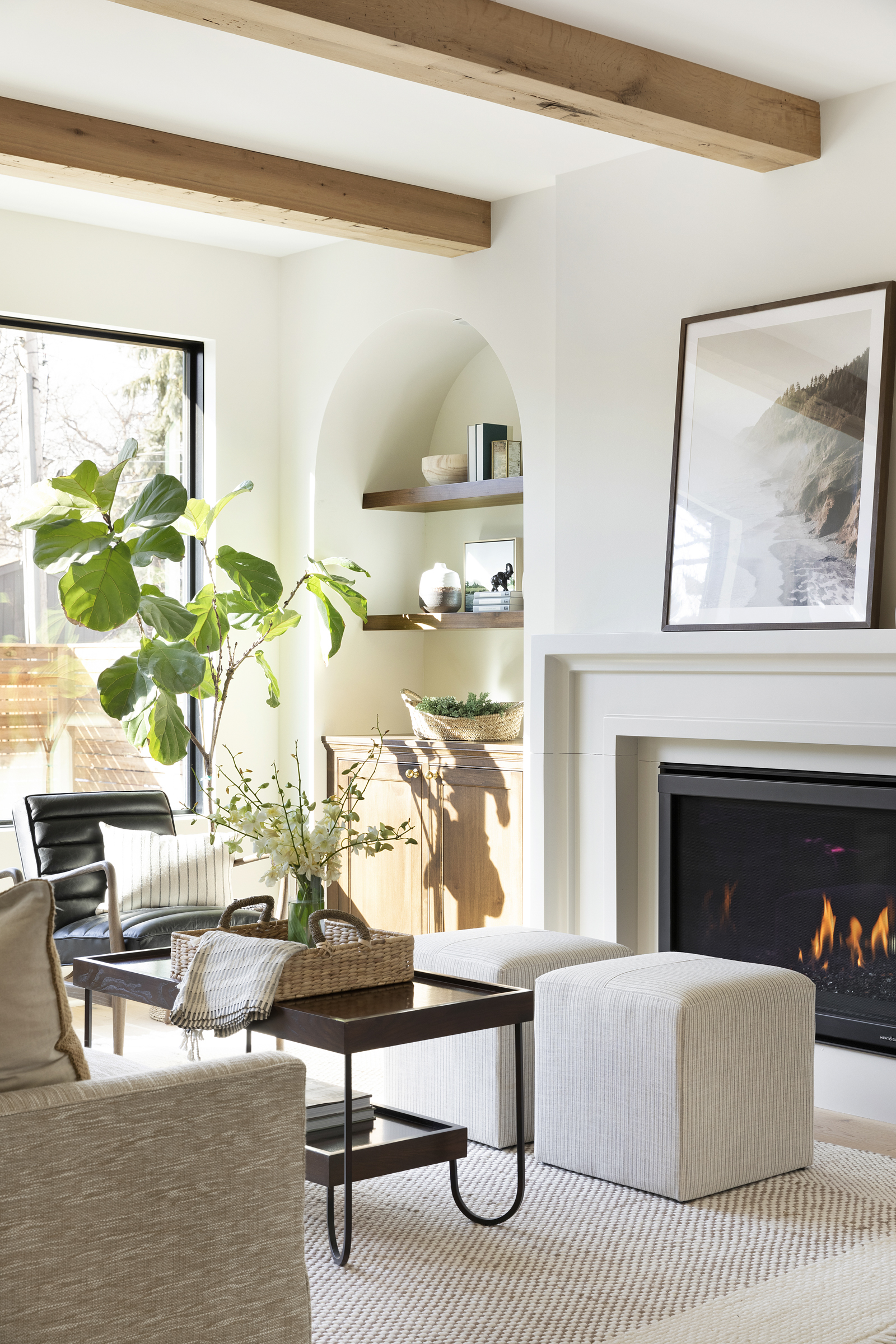This photograph depicts a cozy, modern living room dominated by soft ivory and beige tones. The room features a gas fireplace framed in black, with orange flames dancing invitingly inside. A sleek white mantle above the fireplace supports a tall, shiny black-framed photograph. In front of the fireplace are two beige ottomans on a beige rug, alongside a gray set of cubes, enhancing the room's welcoming atmosphere.

Three rectangular wooden beams traverse the ceiling, adding a rustic charm. To the left of the fireplace is an arched built-in bookshelf with cupboards at the bottom, showcasing books, pictures, and decorative pots. A large window allows natural light to flood the space and hosts a big, green plant in a pot, accentuating the serene ambiance.

Furnishings include a tan-colored couch and a black leather chair with a beige pillow accented with tan stripes. Centrally positioned is a dark wood coffee table with distinctive J-shaped metal legs, featuring a wicker basket with a beige hand towel. The room’s overall layout, with its modern yet country-style design, conveys a staged but homey feeling, perfect for relaxation.